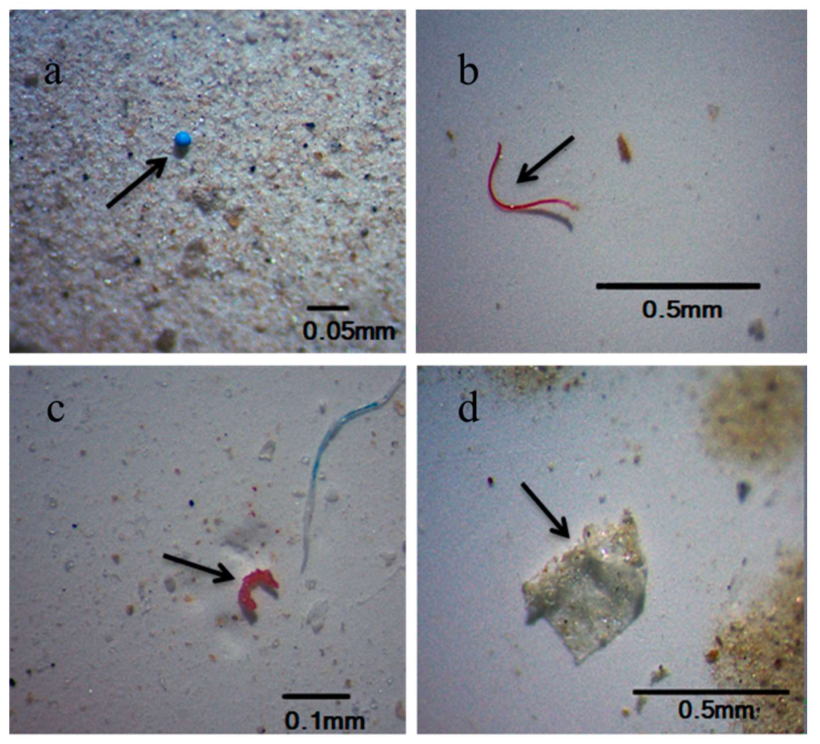The composite image is arranged in a 2x2 grid of four square panels, divided by white borders, suggesting scientific annotation. 

### Panel Descriptions:
- **Top Left (Label: A):** 
  - Features: A small black letter "A" in the top left corner.
  - Imagery: Grainy, sand-like background with a prominent small blue sphere.
  - Annotation: A black arrow points upward and to the right, directing attention to the blue sphere.
  - Scale: At the bottom right, a black horizontal line labeled "0.05 mm" provides scale.

- **Top Right (Label: B):**
  - Features: A small black letter "B" in the top left corner.
  - Imagery: Light gray surface with a sparse scattering of colored specks.
  - Annotation: A black arrow points downward and to the left, toward a red line that extends leftward before curving right, with a small gray line protruding beneath it.
  - Scale: At the bottom right, a black horizontal line labeled "0.5 mm" provides scale.

- **Bottom Left (Label: C):**
  - Features: A small black letter "C" in the top left corner.
  - Imagery: Predominantly white background with lightly colored specks.
  - Annotation: A black arrow points to the right and slightly downward, highlighting a semicircular red shape. Above it, a long blue object moves up and to the right.
  - Scale: At the bottom right, a black horizontal line labeled "0.1 mm" provides scale.

- **Bottom Right (Label: D):**
  - Features: A small black letter "D" in the top left corner.
  - Imagery: White background interspersed with brown, sand-like grains, particularly evident at the corners.
  - Annotation: A black arrow points downward and to the right, focusing on a silvery white object with some sand grains on it.
  - Scale: At the bottom right, a black horizontal line labeled "0.5 mm" provides scale.

Overall, the structured grid layout and detailed annotations with arrows and scale markers suggest the image is part of a scientific study or analysis.